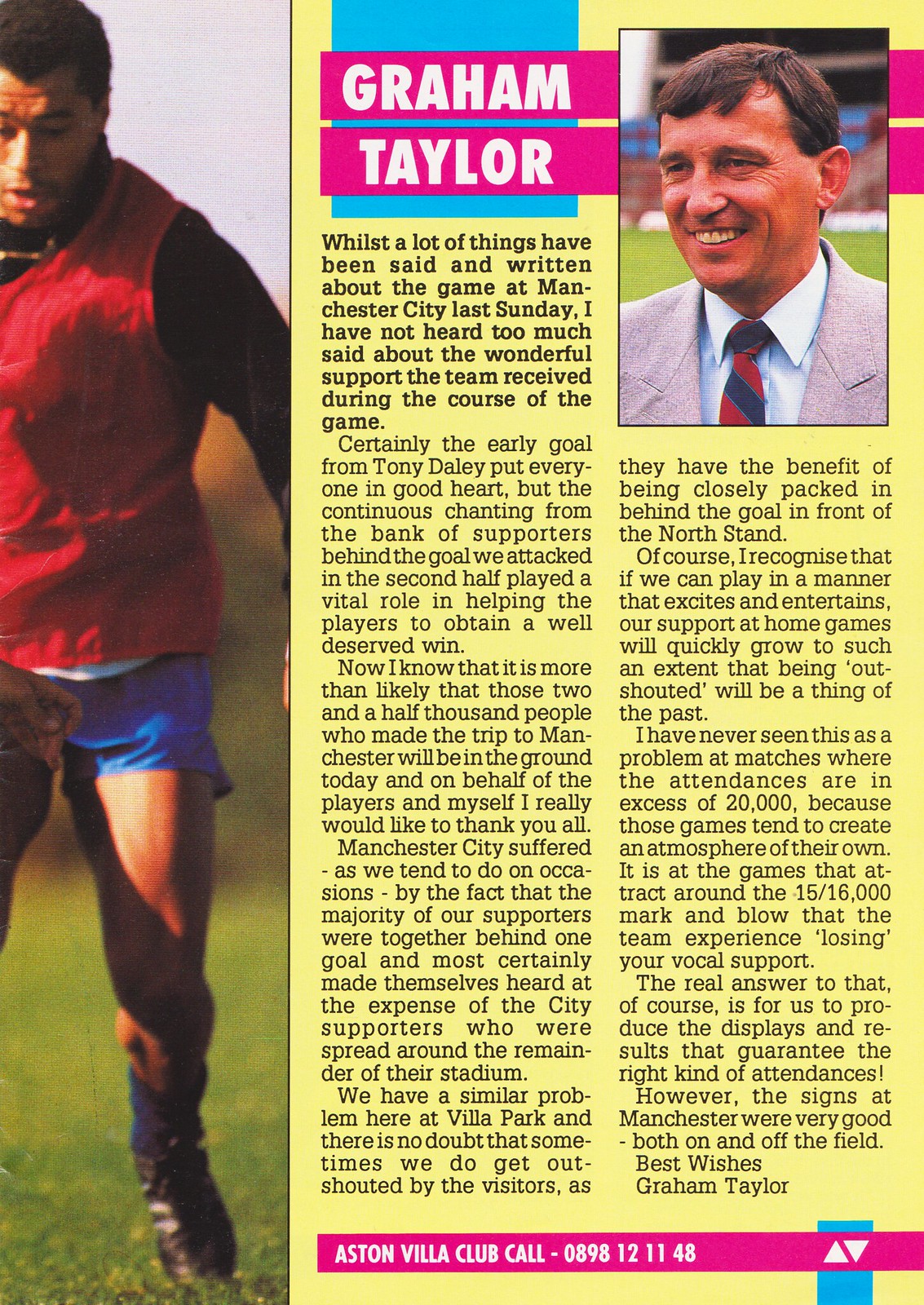This image captures a page from an English football magazine, divided into three vertical sections. On the left, there's a vertical banner featuring an action shot of a soccer player in practice, wearing a black long-sleeved shirt under a red vest with blue shorts, set against a grassy field. The middle and right sections contain a lengthy article under a yellow background. At the top of the article, there's a headshot of a man in a light-colored suit with a red and blue tie, and to the left of this photo, it reads "Graham Taylor." The article discusses a recent football game held in Manchester City, highlighting the remarkable support the team received, especially noting the early goal by Tony Daly and the continuous chanting from supporters, which played a crucial role in securing a well-deserved win. At the bottom of the page, a pink rectangle lists the contact information for the Aston Villa Club, with the number 090-898-1211-48.